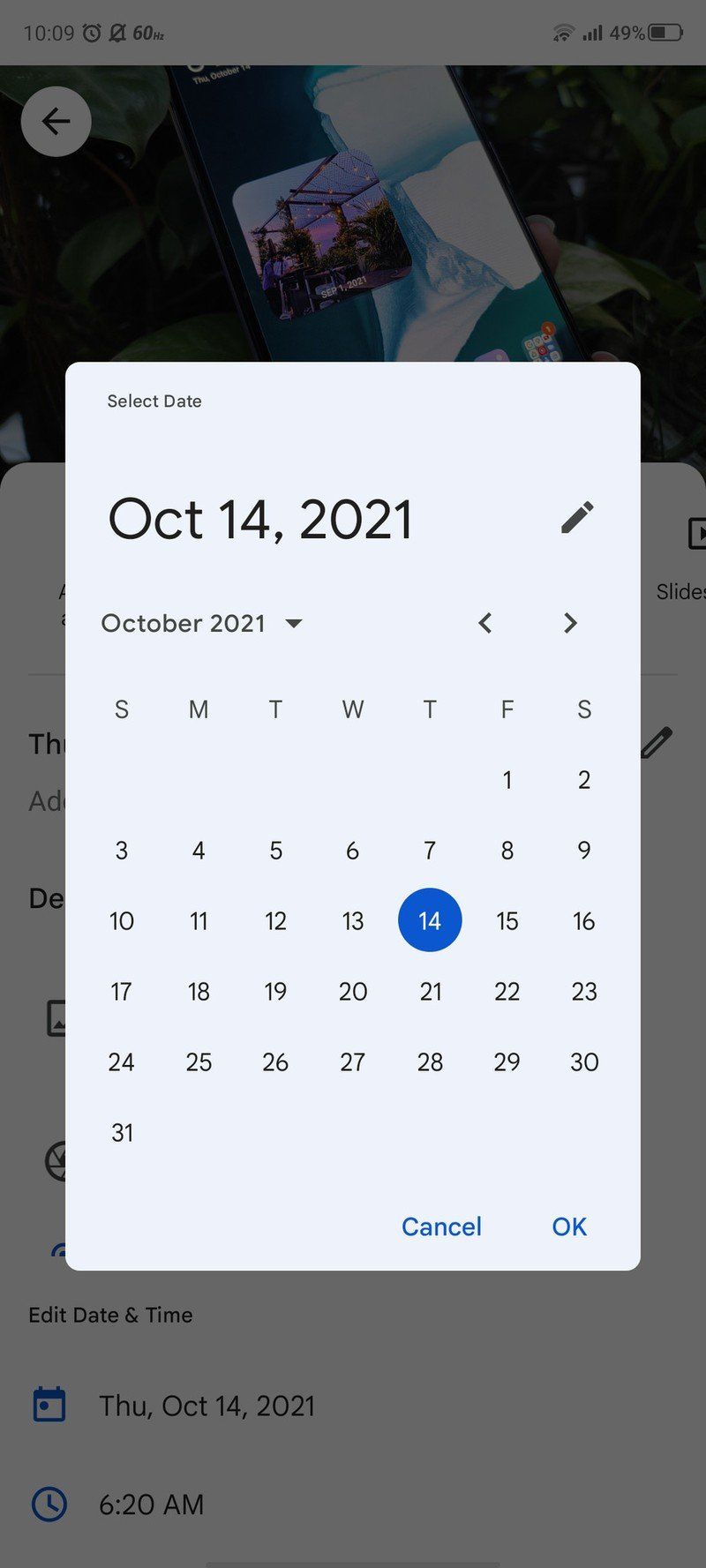A screenshot captures a cell phone display showcasing a date selection pop-up window from October 14th, 2021. The pop-up window is primarily white. In the upper left corner, the text "Select Date" appears in a small black font. Directly beneath this, the date "October 14, 2021" is displayed prominently in a larger black font, accompanied by a pencil icon to its right, signifying the ability to edit. Below, "October 2021" is indicated in a smaller font along with a drop-down arrow, enabling month selection. Adjacent to this text are navigational arrows for scrolling left or right through the calendar. The calendar grid features the days of the week abbreviated as "Sun, Mon, Tue, Wed, Thu, Fri, Sat." The date "14" is distinctly circled, highlighting it within the numerical days of the month.